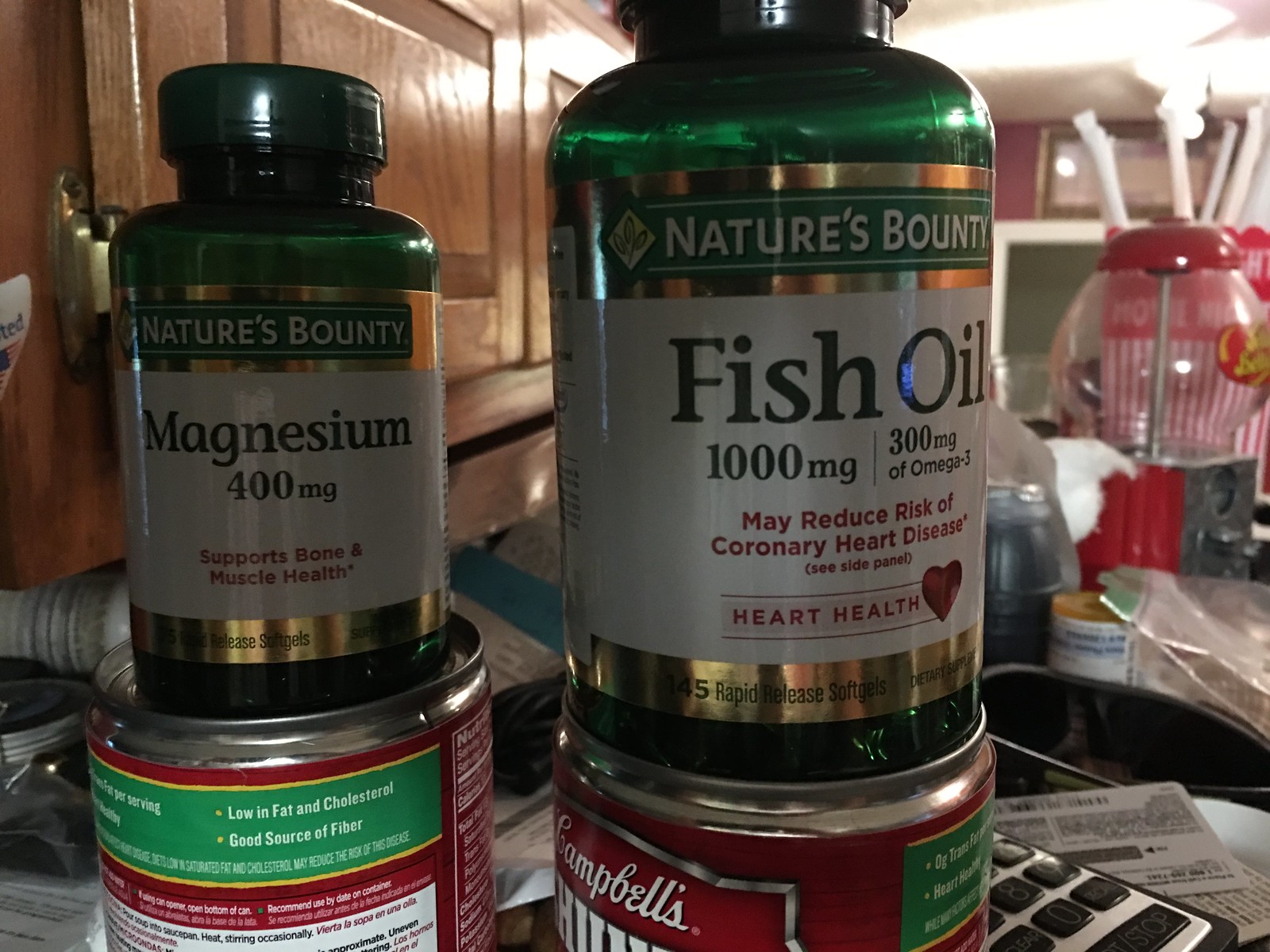The image captures a variety of items arranged indoors. Prominently placed in the front right corner is a bottle labeled "Fish Oil." The label includes the brand name "Nature's Bounty" at the top, followed by the dosage "1000 MG." Adjacent to this, it specifies "300 MG of Omega-3." Further down, the label mentions, "May Reduce Risk of Coronary Heart Disease* (See side panel)," and emphasizes "Heart Health" accompanied by artwork of a red heart. The bottle itself is predominantly green. To the left of the Fish Oil bottle, there's another bottle also branded "Nature's Bounty," featuring the label "Magnesium, 400 MG." The image is rich in detail, showcasing the carefully printed text and vibrant colors of the packaging.